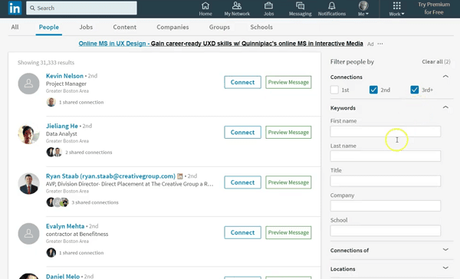Screenshot Description:

The screenshot captures an interface with a teal-themed design and a rich array of features. At the top, embedded in a navy blue header, several interactive elements can be seen. Starting from the left, there is a teal-colored box labeled "in" followed by a white search bar. Continuously to the right within the navy blue section, there are several navigation options including "Home," "My Bookmark," "My Profile," "Sales Managing," "Notifications," "Me," and "Work."

Further in this section, additional functionalities are listed such as "Try Production for Free." Below these menu options, there are categorized tabs starting with "All," highlighted with teal underlines, followed by "People," "Jobs," "Contact," "Companies," "Groups," and "Schools."

The main content area displays information pertaining to a digital course touting "Online MS in UX Design," advertising career-ready skills through "Quinn PX Online MS in Interactive Media." Below this, profiles of various professionals are featured, including Kevin Nelson, a Project Manager; Huling Yi, a Data Analyst; Ryan Staub, an AVF Division Director at Direct Placement for The Creative Group; and Evelyn Mehta, a Contractor at Bond Fitness.

On the far right, there is a filter section labeled "Filter People By." Current applied filters include "Connections," with "Second" and "Third" degree connections checked. A notification icon, represented by a yellow circle with the number '1,' is notable towards the end.